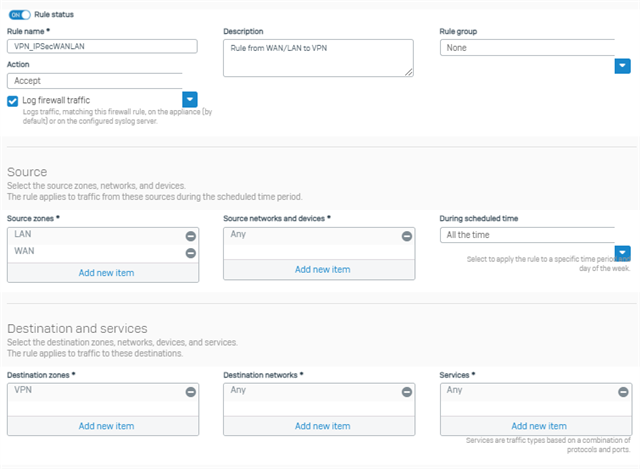**Detailed Description of the Online Form Interface**

The image depicts a landscape-oriented, rectangular online form interface, commonly seen on computer screens, especially laptops. The background is predominantly white, with thin borders at the top and bottom of the interface, while the sides remain borderless. 

At the very top of the image, a thin, light-gray line outlines the upper border. Positioned immediately below this line, in the left corner, is an elongated oval shape with a teal-blue background. Within this shape, the left side contains the white text "on," and a white circle is positioned to the right, illustrating an activated toggle switch. To the right of this toggle, the black text reads "Rule Status."

Below this top section, the form is divided into various fields arranged in three columns. Here's a detailed breakdown:

### Left Column:
- **First Field ("Rule Name *"):**
  - Header: "Rule Name *"
  - Content: "VPN_IP" followed by additional letters
- **Second Field ("Action"):**
  - Header: "Action"
  - Content: "accept"
  - Beneath this field: 
    - A blue box with a white checkmark
    - Text: "Log firewall traffic"
    - A blue box with a downward-facing arrowhead, indicating a dropdown menu
    - Two lines of small text: "log in traffic, ..." (trailing off)

### Middle Column:
- **Field ("Description"):**
  - Header: "Description"
  - Content: "rule from WAN/LAN to VPN"
  - Bottom-right corner has diagonal lines for resizing the field

### Right Column:
- **Field ("Rule Group"):**
  - Header: "Rule Group"
  - Content: "none"
  - Below this field: 
    - A blue square with a white downward-facing arrowhead

### Middle Section:
- A light gray rectangular background spans across the middle.
  - Text within it: 
    - "Enlarge font source"
    - Lines below: "Select the source zones, networks, and devices." 
    - Continued text: "The rule applies to..."

### Bottom Section (Three Fields):
- **Left Field ("Source Zones *"):**
  - Header: "Source Zones *"
  - Content: 
    - Row 1: "LAN"
    - Row 2: "WAN"
    - Row 3: Centered blue text: "add new item"
  - Right side of rows 1 & 2: gray circles with white horizontal lines (delete options)

- **Middle Field ("Source Networks and Devices *"):**
  - Header: "Source Networks and Devices *"
  - Content:
    - Row 1: "any"
  - Below: Centered blue text: "add new item"
  - Right side of row 1: gray circle with white horizontal line

- **Right Field ("During Scheduled Time"):**
  - Header: "During Scheduled Time"
  - Content: "all the time"

### Bottommost Section:
- Gray background labeled "Destination and Services"
  - Lines below: 
    - Text: Additional details (incomplete)
  
- **Three Fields Below ("Destination Zones *", "Destination Networks *", "Services *"):**
  - **Left Field ("Destination Zones *"):**
    - Header: "Destination Zones *"
    - Content:
      - Row 1: "VPN"
      - Row 2: Center blue text: "add new item"
  - **Middle Field ("Destination Networks *"):**
    - Header: "Destination Networks *"
    - Content:
      - Row 1: "any"
      - Row 2: "add new item"
  - **Right Field ("Services *"):**
    - Header: "Services *"
    - Content:
      - Row 1: "any"
      - Row 2: "add new item"
  
  - Right side of each row: gray circles with white horizontal lines

All fields are horizontally and vertically aligned, featuring headers positioned directly above the input areas. The form maintains a clean, methodical structure, emphasizing usability with easily identifiable input areas and clear labels.